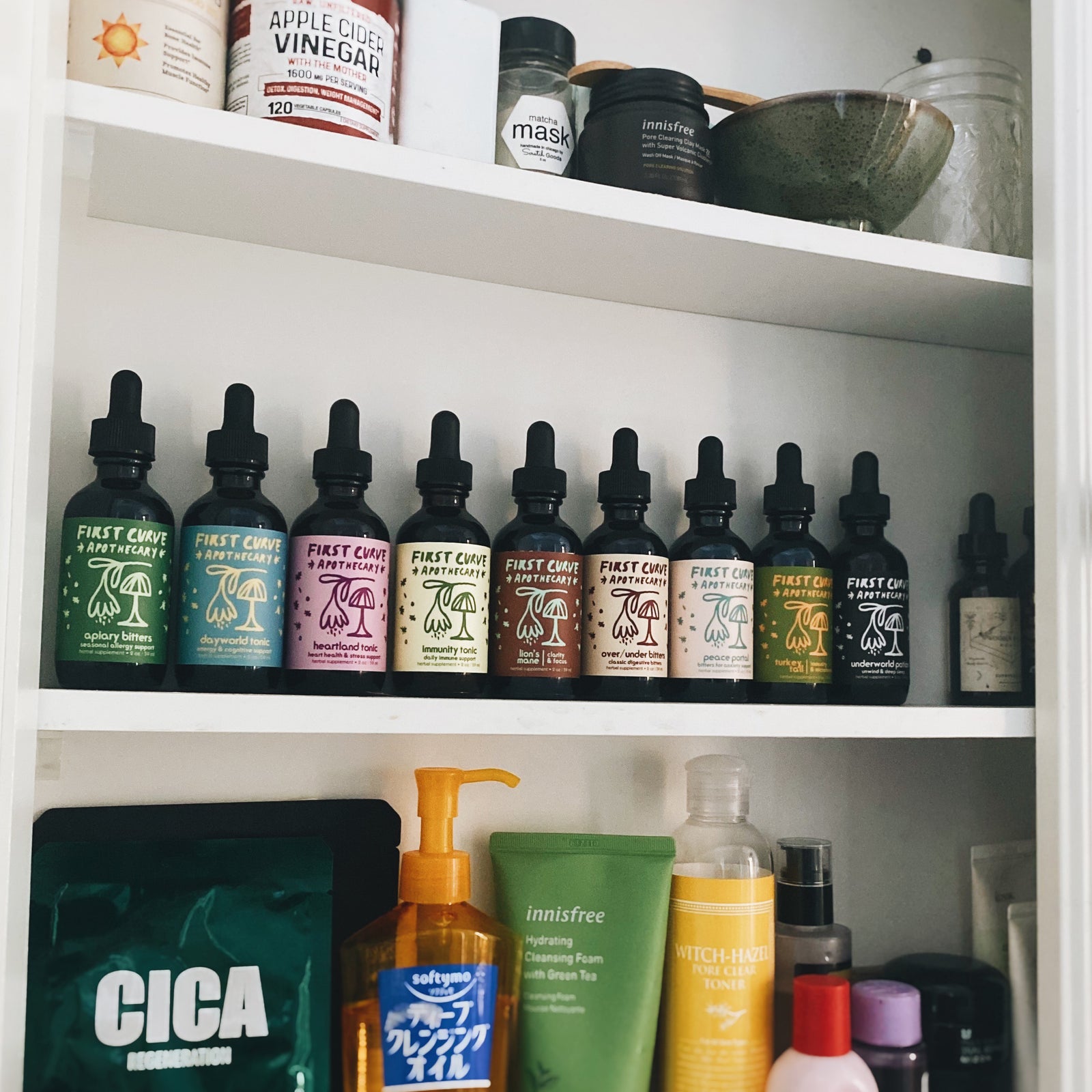This detailed photograph shows the interior of a white cabinet with three shelves, each brimming with various beauty products. The top shelf features an array of items, including a large bottle of apple cider vinegar with black text specifying its composition and a face mask jar labeled "muc-a-mask." Next to these are a green mixing bowl and a transparent mason jar. The middle shelf showcases ten bottles from the First Curve Apothecary line, each adorned with a unique label in colors like green, pink, beige, cyan, and black, each featuring a mushroom and plant design. The bottom shelf contains a variety of bottles and tubes, including a hydrating cleansing foam, an olive-green tube labeled "insafree," a multitude of soap bottles, and other partially visible lotion bottles with tops in various colors—orange, black, red, purple, and blue. All products collectively present a well-organized yet diverse beauty collection.